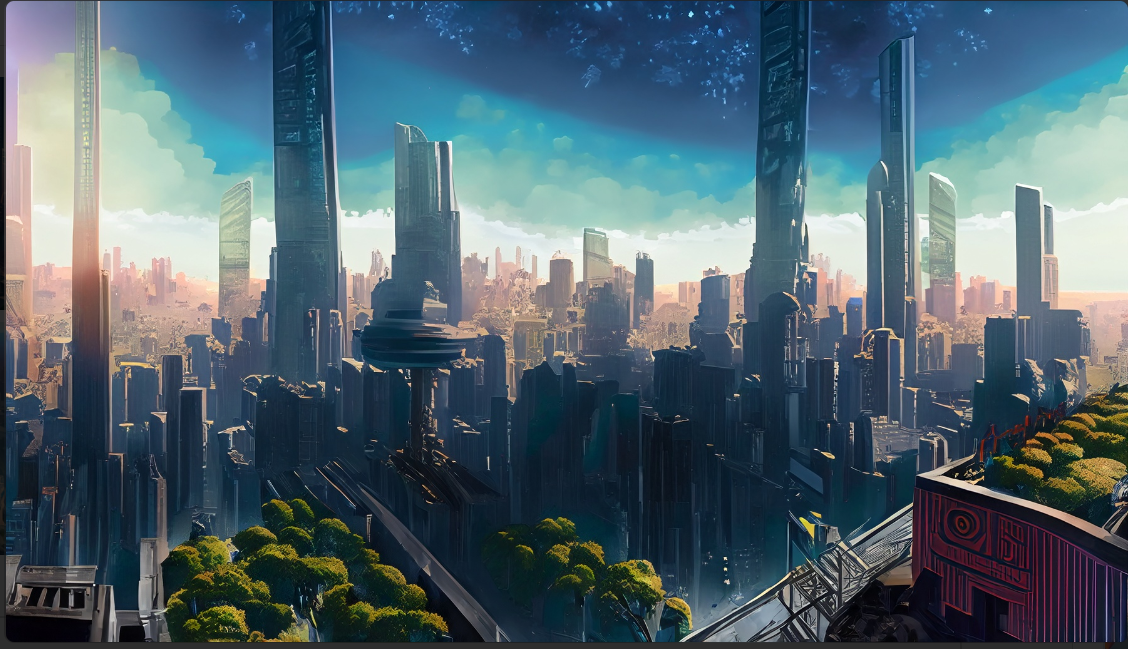The image is a highly detailed digital or AI-generated artwork depicting a futuristic city. The cityscape is densely packed with tall, skinny skyscrapers of varying heights, many of which extend beyond the top of the frame. The buildings in the foreground are predominantly dark blue, lending a sleek, modern aesthetic typical of future cities. In the bottom section of the image, smaller skyscrapers and a scattering of tall trees with large green canopies add a natural element to the scene. Notably, there is a short red building with green bushes or shrubbery on its roof situated in the bottom right-hand corner. The sky above the city transitions through multiple shades of blue, from a darker blue at the top to lighter shades towards the horizon, where it meets an area of white. The clustered arrangement of the buildings emphasizes the high-density nature of the city, contrasting with the green spaces interspersed throughout.